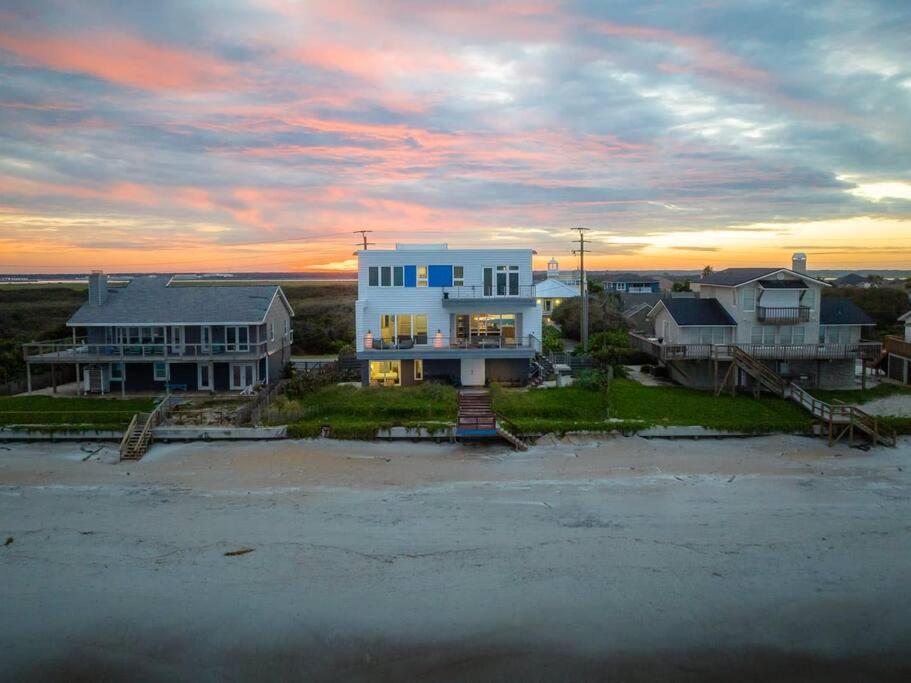The photograph depicts a scenic beachside with three distinct houses aligned along the shoreline. The foreground features sand stretching towards the bottom half of the image, suggesting the picture was taken from the beach. 

The central focus is a white, three-story house. This house has a wooden staircase leading up to the backyard patio area, complete with a combination of white double doors and glass sliding doors. The structure also features blue shutters and appears to be constructed from paneling and possibly some bricks at the base. On either side, it is flanked by two additional houses. 

The house on the left is a two-story structure with gray siding, white-framed windows, a gray roof, and a second-story deck. The house on the right is also two stories, distinguished by its beige color and dark roof, with a deck and stairs descending to the beach. Both houses appear well-maintained despite their simple materials.

In front of these houses, there is vivid lime green grass leading out to the sandy beach. Above, the sky displays a beautiful sunset with an orange hue blending with dark blue clouds, casting a serene and picturesque backdrop to the scene.